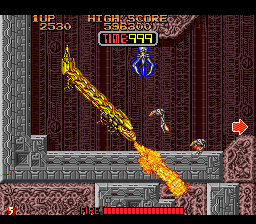This screenshot from an older video game features a golden forearm or weapon emitting a lateral flame directed to the left. The graphics are notably dated, with a background showcasing mauve, textured vertical stripes and an ornate cement wall on the left. At the bottom of the screenshot, text and numerical information are displayed: "High Score" at 5596300, and "Time" set to 999 in yellow within a red oval. In the upper left corner, "1UP" is marked at 2530, accompanied by an orange arrow pointing right. A gauge labeled "Fire" is positioned at the bottom, red on the far left, with the number 5 in white encircled in red at the base. The wall features a couple of characters and a small, blurry, floating object, possibly another weapon. Centrally, a creature resembling a spider or scorpion hangs from the ceiling, adding an element of suspense to the game scene.